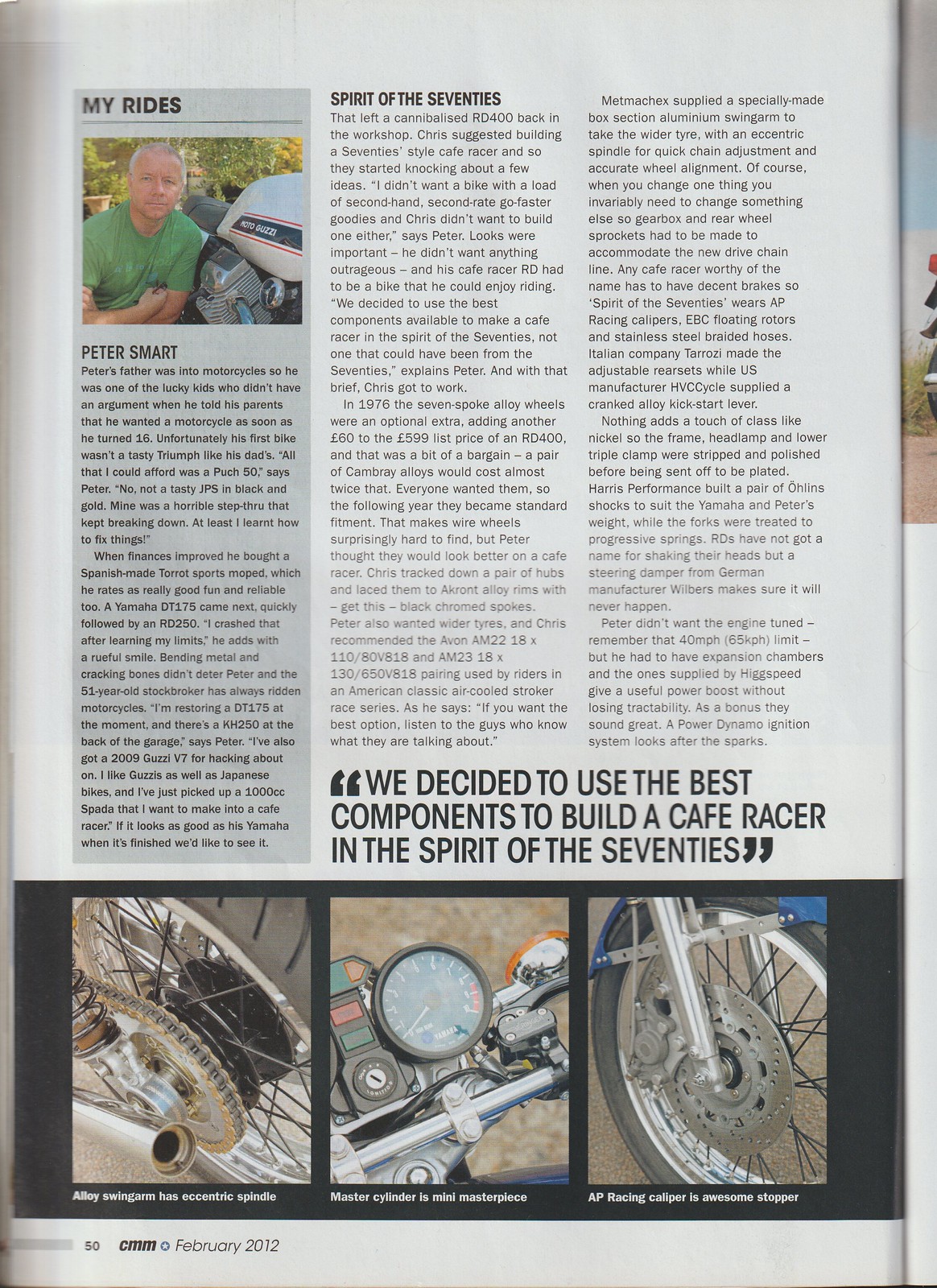This interior magazine page dedicated to the theme "My Ride" showcases an exclusive feature on Peter Smart and his motorcycle. The top portion of the page prominently displays a photograph of Peter Smart, dressed in green, taking a picture beside his motorcycle. The accompanying text, tagged as "My Ride," introduces Peter Smart and delves into his narrative across two columns of the article.

At the conclusion of the main article, in bold black text, it reads: "We decided to use the best components to build a cafe racer in the spirit of the 70s." This statement captures the essence of the motorcycle's vintage inspiration.

Beneath the article, the page features a detailed close-up series of various motorcycle parts. On the left is an image showcasing the bike wheel with visible chain links. The center photograph highlights the master cylinder, accompanied by a blue gauge near the ignition switch area, described as a "mini masterpiece." The final image on the right displays the AP Racing caliper, touted as an "awesome stopper."

The article and images together emphasize the meticulous selection of components to achieve a retro-style cafe racer, embodying the aesthetic and mechanical spirit of the 1970s.